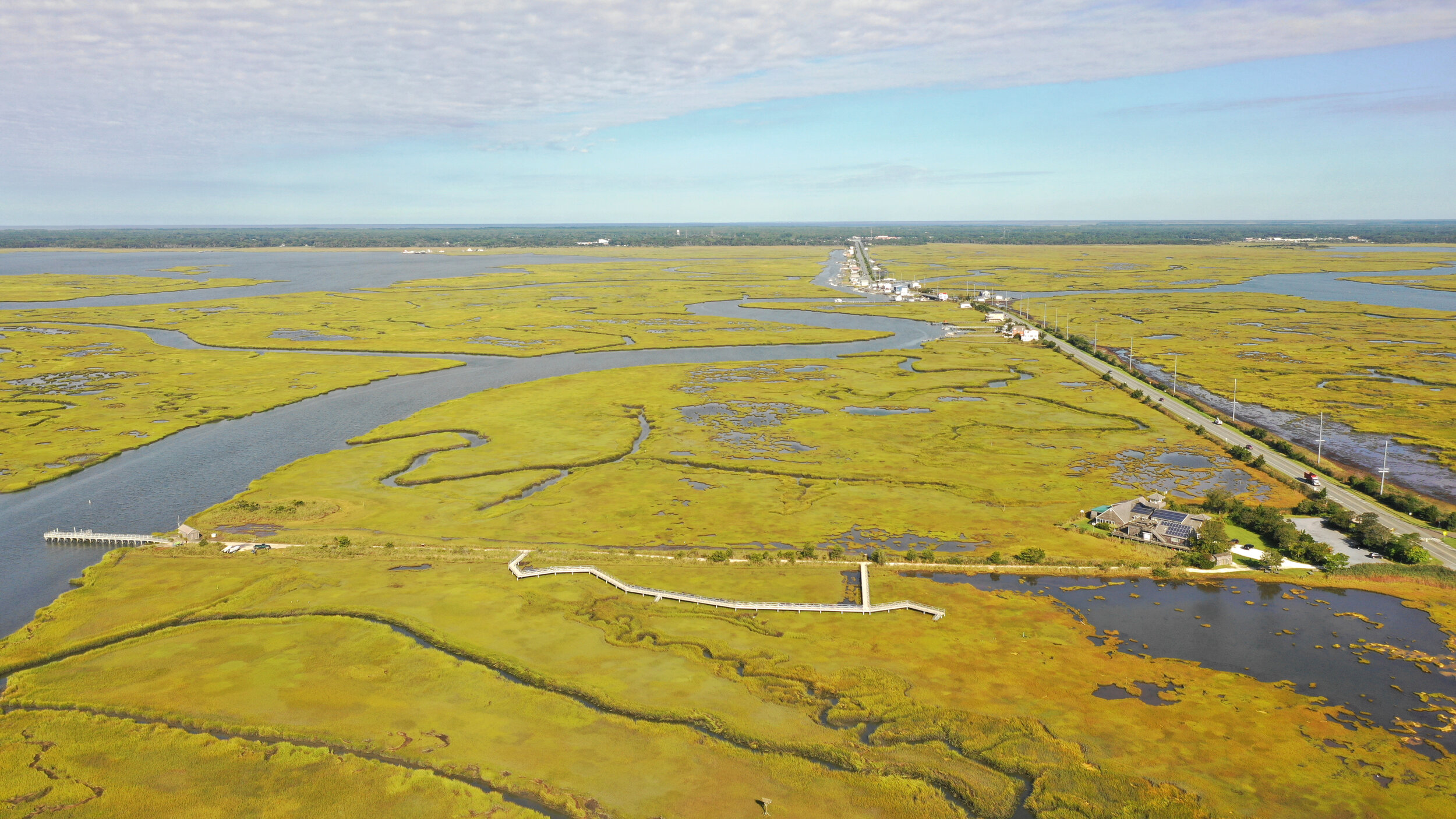The image depicts a vast, flat landscape, reminiscent of the Everglades, characterized by swampy terrain and extensive wetland. The right third of the image showcases a two-lane road cutting through this swampy area, adorned with light yellow-green floating plants that suggest a rich, aquatic environment. Rivulets of water weave through the vegetation, hinting at pathways used by pontoon boats or similar watercraft navigating the marsh-like setting. 

Midway into the frame, there's a small community of houses clustered near the road, around 200 feet away from it, with a dock extending out to the river on the left side of the photo. The wetland is interspersed with patches of what seems to be dead grass or possibly a yellow film on the water's surface, suggesting an area either of swamp vegetation or an algae bloom. 

In the distant background, the road appears to lead towards the horizon where either the ocean or another large body of water meets the sky. The upper portion of the image features a clear, light blue sky with scattered white clouds, accentuating the bright, sunny ambiance of the scene. A bridge can be seen further down the road, crossing over another section of water, solidifying this setting as a tranquil yet intricate landscape where natural waterways and human infrastructure coexist.